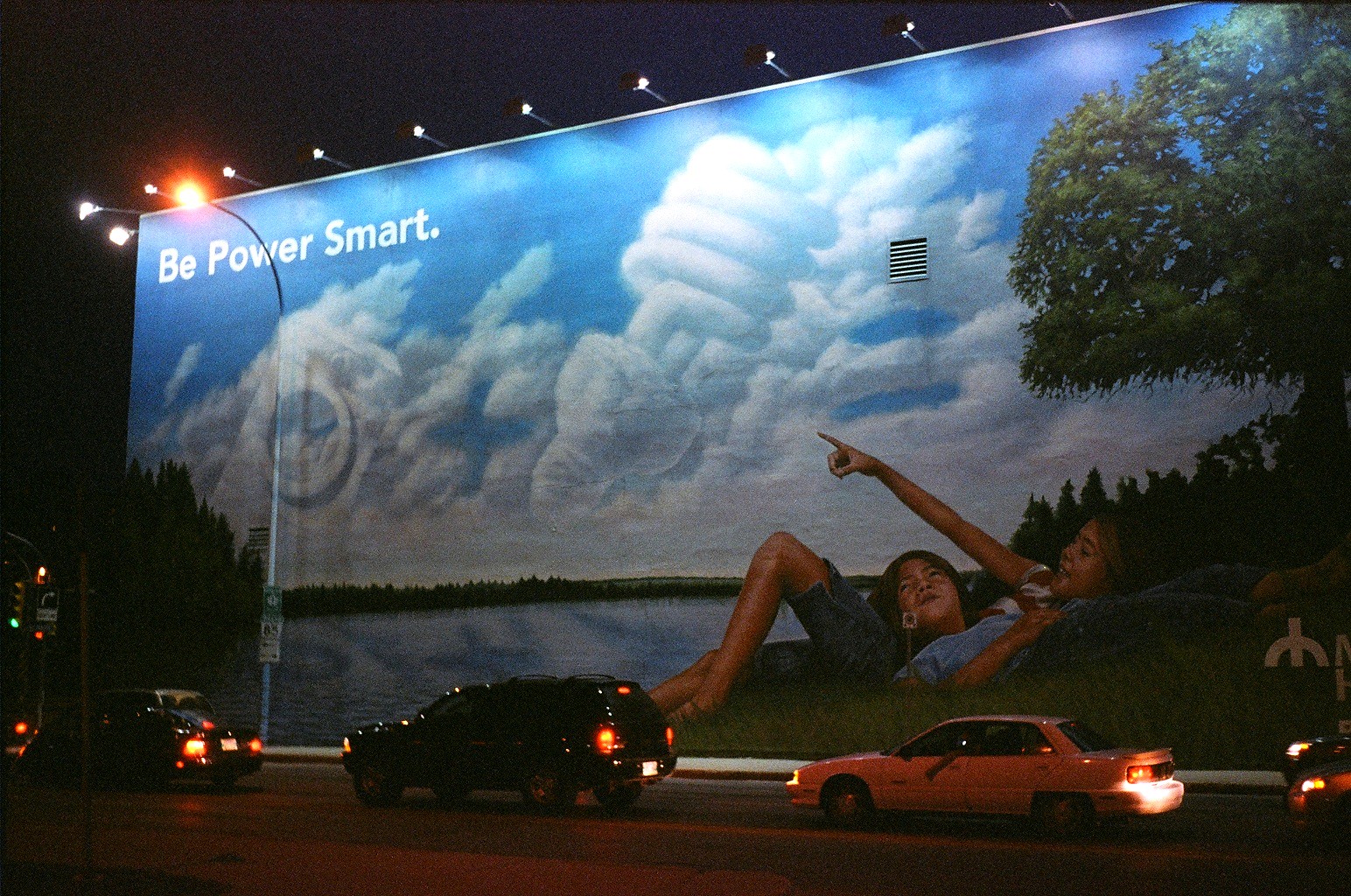This photograph, captured in a widescreen format, depicts a nighttime scene at a busy intersection. The frame is dominated by a row of cars, their brake lights glowing a vivid red, halted at a traffic light. There are three visible vehicles, and a fourth one on the right side, where only its front headlights are apparent. Additional vehicles are scattered around the intersection, suggesting a moment of pause in the city's ceaseless traffic flow.

The background is graced by an imposing billboard that stretches from the ground to the top of the frame. This massive advertisement features two women lying on a grassy expanse. One woman, with her head resting on the other's lap, is pointing towards the sky. The sky above is artistic, adorned with clouds and several disembodied hands. One hand holds a pointing finger, while another grips onto an LED light bulb.

On the upper left side of the billboard, a message in crisp text declares, "Be Power Smart," urging viewers to consider energy efficiency. The scene, with its intricate play of lights and the contrasting stillness of the advertisement, creates a captivating snapshot of urban life and commercial messaging.